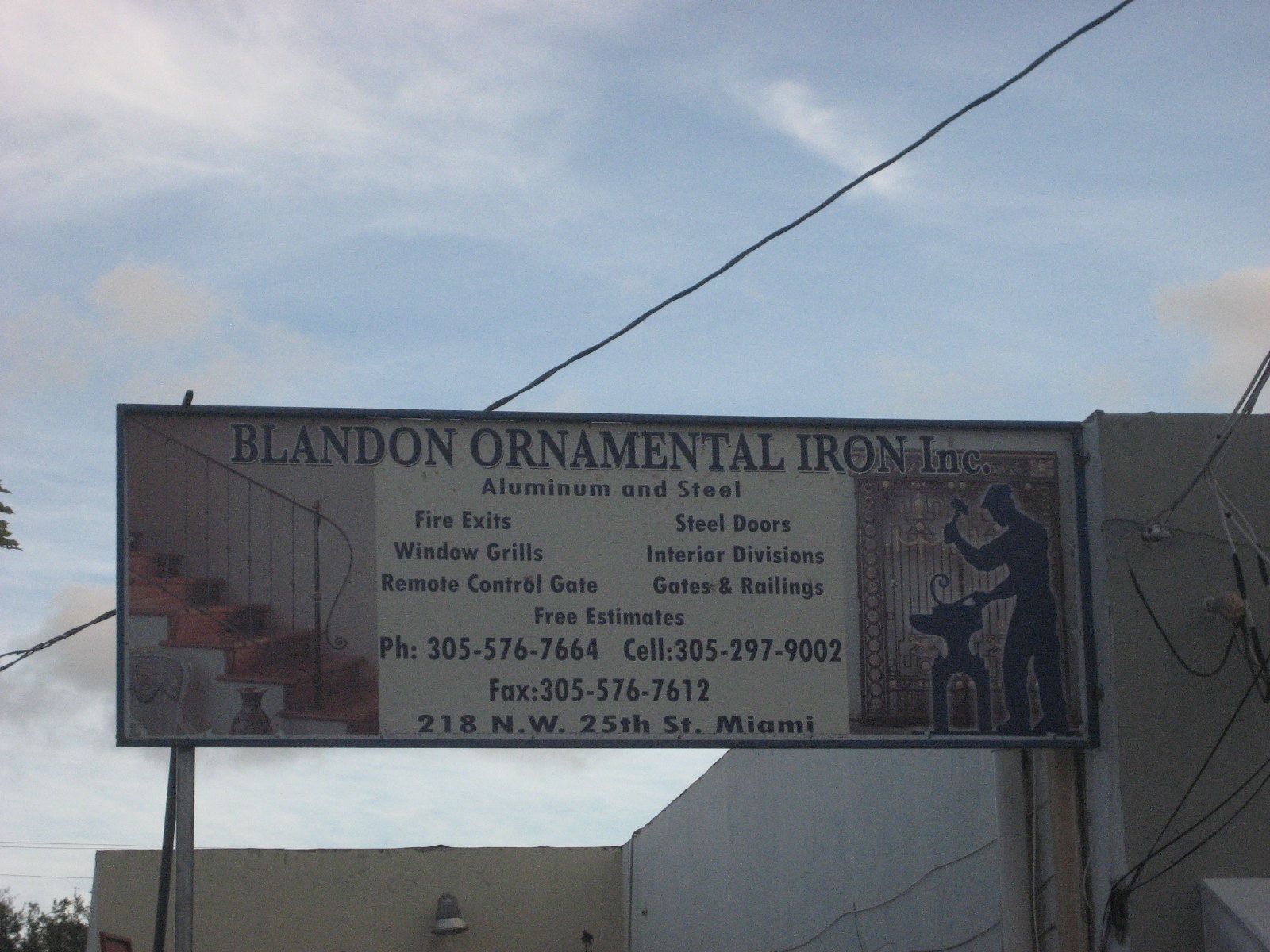In this vibrant outdoor photograph taken during the daytime, the sky dominates the upper portion with bright blue hues interspersed with feathery white clouds. Stretching diagonally from the upper right to the lower left is a power line, adding an industrial touch to the scene. Central to the image is a large, horizontally aligned, rectangular sign for Blandon Ornamental Iron Incorporated, displayed in bold black, all-capital letters. Below the company name, the services listed include "Aluminum and Steel," with two columns detailing specific services: on the left, "Fire Exits, Window Grills, Remote Control Gates," and on the right, "Steel Doors, Interior Divisions, Gates and Railings." Centered beneath these columns is the enticing offer of "Free Estimates," followed by the contact information: "PH 305-576-7664, Cell 305-297-9002, Fax 305-576-7612," and the address, "218 NW 25th Street, Miami."

Flanking the text, on the left side, there is an illustrated example of a staircase with ornate iron railings, while on the right, a blacksmith is depicted hammering an anvil, signifying craftsmanship. Below the sign, a beige and brown stone building with an overhead light or spotlight peeks into the frame, enhancing the industrial ambiance of the setting. This detailed portrayal showcases the blend of artistic ironwork and practical services offered by the company, set against the expansive, cloud-dotted sky.